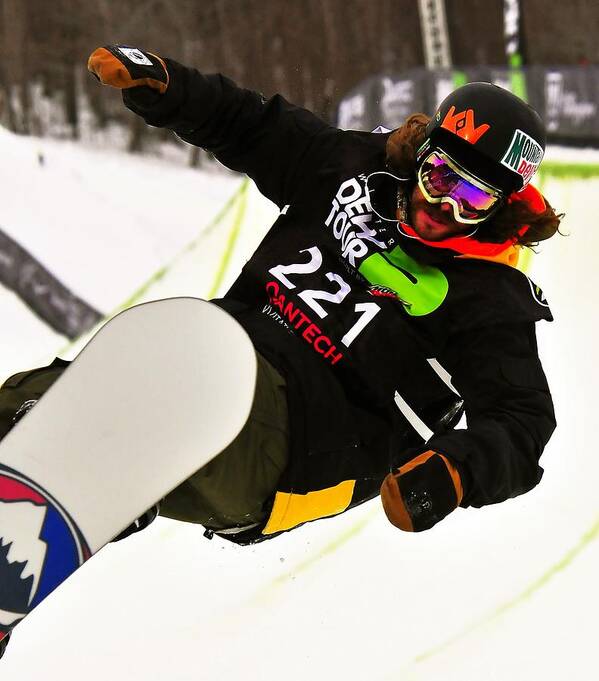The image captures a dynamic action shot of a snowboarder, identifiable as a Caucasian male with a distinctive appearance. He is airborne over a snow-covered half-pipe, its sharply defined walls adorned with green stripes. In the background, a serene landscape of snow and trees contrasts starkly with the action.

The snowboarder boasts a rugged look with long, wavy brown hair, a brown mustache, and beard. His outfit consists of a black helmet branded with "Mountain Dew" on one side and a crown on the other. He wears a heavy black, long-sleeved jersey featuring the number 221 in white text and "Kantech" in red beneath it. His jersey is complemented by brown and black gloves, possibly North Face, and a red muffler around his neck. Olive green snow pants complete his attire.

His snowboard is white with red and blue markings on the bottom, featuring a graphic of a mountain with a white top and gray bottom. The snowboarder is in mid-jump, angled with his legs to the left and bending his body to the right, showcasing his skill and the thrill of the competition. The detailed elements of his attire and equipment, along with the backdrop, encapsulate the excitement and intensity of the snowboarding event.